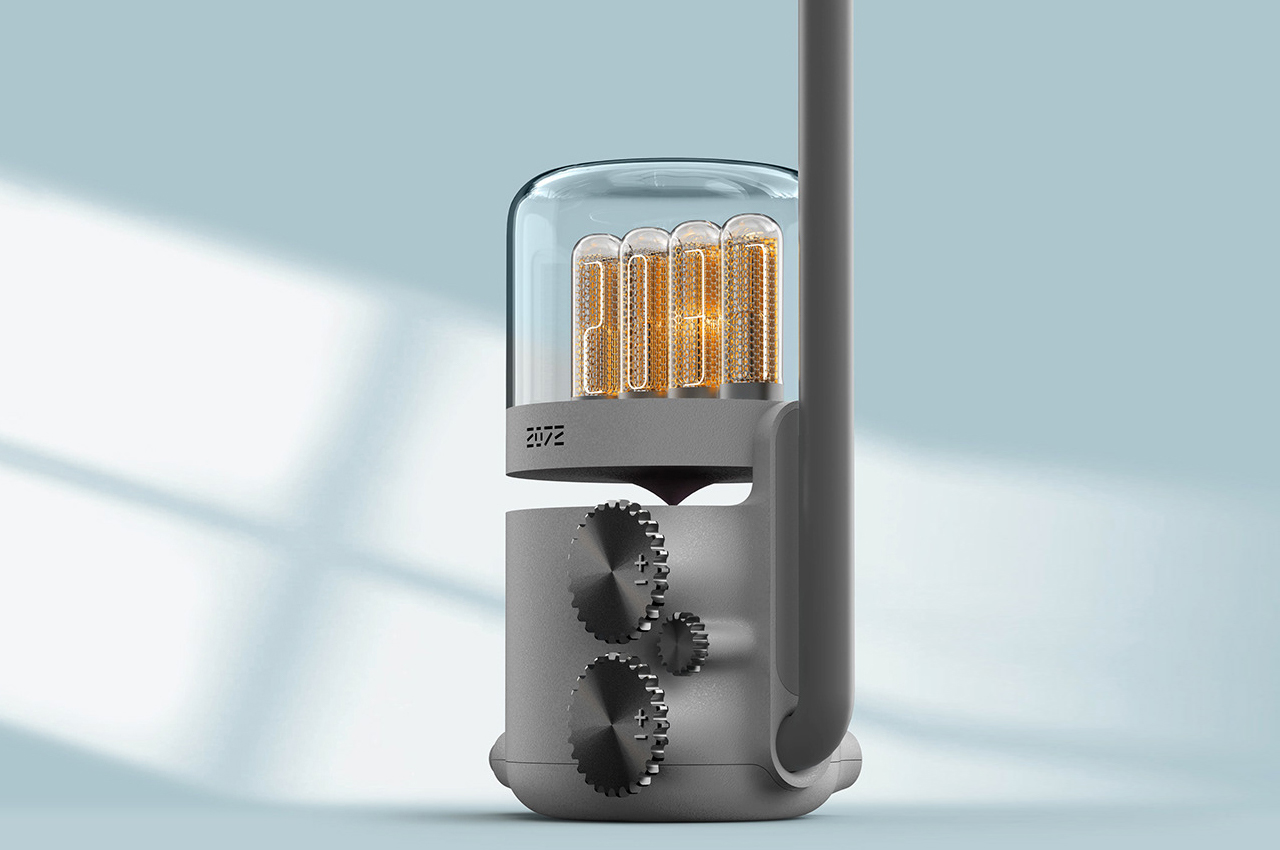The photograph features a distinctive mechanical-technological device set against a light blue backdrop, which displays reflections of window sills and light. Central to the image is a gray, walkie-talkie-like apparatus, notable for its matte charcoal black body and clear glass top section. This transparent upper part houses four illuminated tubes, reminiscent of vintage vacuum tubes seen in guitar amplifiers, glowing in a golden hue. Inscribed within the glass tubes, numbers '2037' are visible in a white light. The front of the device's gray chassis bears the number '2072,' and it is equipped with three black dials—two large overlapping dials and one smaller one slightly behind. These dials, featuring plus and minus signs, suggest functionality akin to volume control. Additionally, a long gray antenna extends from the right side of the device. The combination of the intricate glass tubes and the sleek gray and black chassis presents an enigmatic yet fascinating piece of technology.